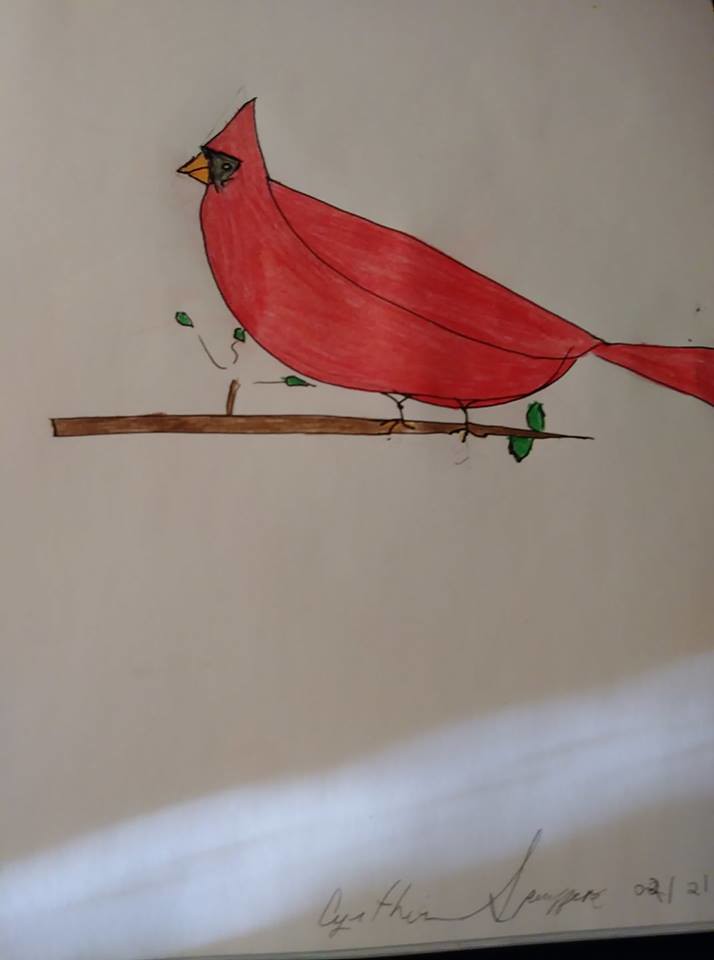This is a simple yet colorful illustration of a cardinal bird perched on a horizontal branch. The bird is primarily red, including its body and tail, with a small pointy crest on its head, and it features an orange or yellow beak. Surrounding the eye area is a distinct black marking. Drawn with swooping lines, the cardinal’s proportions are exaggerated, giving it a large, boat-like body compared to its smaller head and tail. The branch it perches on is depicted with small green leaves and extends horizontally across the upper half of the image, floating with no visible attachment to a tree. The bird clutches the branch with black stick-like legs. The paper appears to be white with a streak of shading or light running diagonally across the bottom portion. In the bottom right corner, there is an artist's signature and the date "February 21," though the signature is not fully legible.